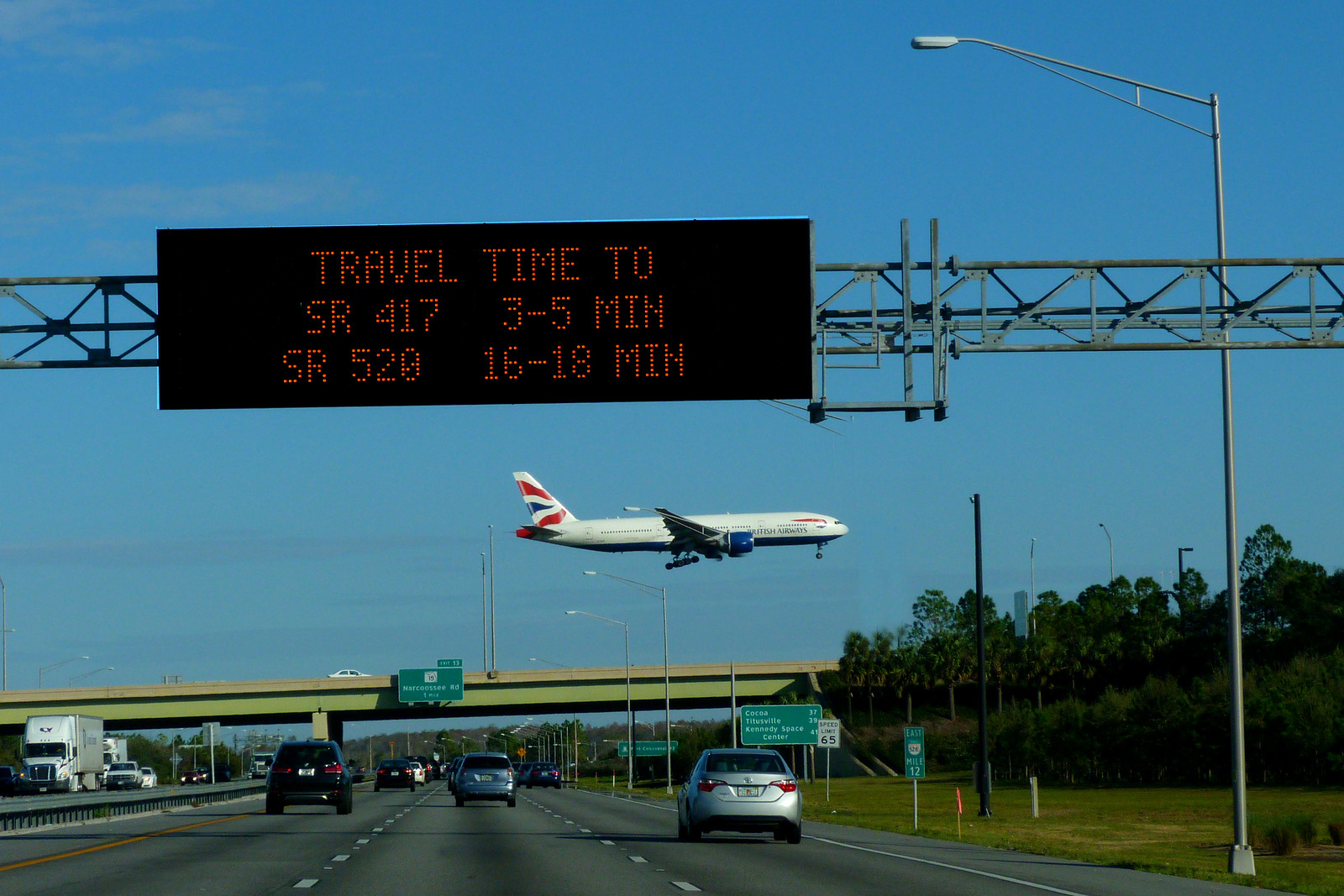This captivating photograph, taken from the driver's perspective, captures a bustling roadway scene beneath a majestic airplane making its descent. The road is divided into two separate three-lane sections by a gray metallic barrier. The three lanes on the right are flanked by those on the left, creating a well-organized flow of traffic. In the rightmost lane, a sleek silver car cruises along, while a striking silver-blue vehicle occupies the middle lane. Farther left, a dark-colored car, potentially dark gray or black, moves away from our view.

Dominating the center-left of the image is an informative road sign displaying travel times to various routes. It reads, "Travel Time 2," followed by "SR-417, 3-5 min" and "SR-520, 16-18 min." This vital information is supported by a horizontal girder-like structure, also gray, that spans the width of the road. 

A towering aluminum light pole rises on the left side of the road, crowned with a street light that likely illuminates the thoroughfare at night. The left edge of the scene is bordered by lush green trees, adding a touch of nature to the primarily urban setting. 

Above all, the photograph features an impressive airplane, white with a tail adorned in red, white, and blue accents, and a visible blue engine. This aerial giant gracefully descends, creating a dynamic focal point that encapsulates the blending of terrestrial travel and aviation. The clear, vivid detail encapsulates the essence of a typical yet extraordinary moment on this well-traveled route.